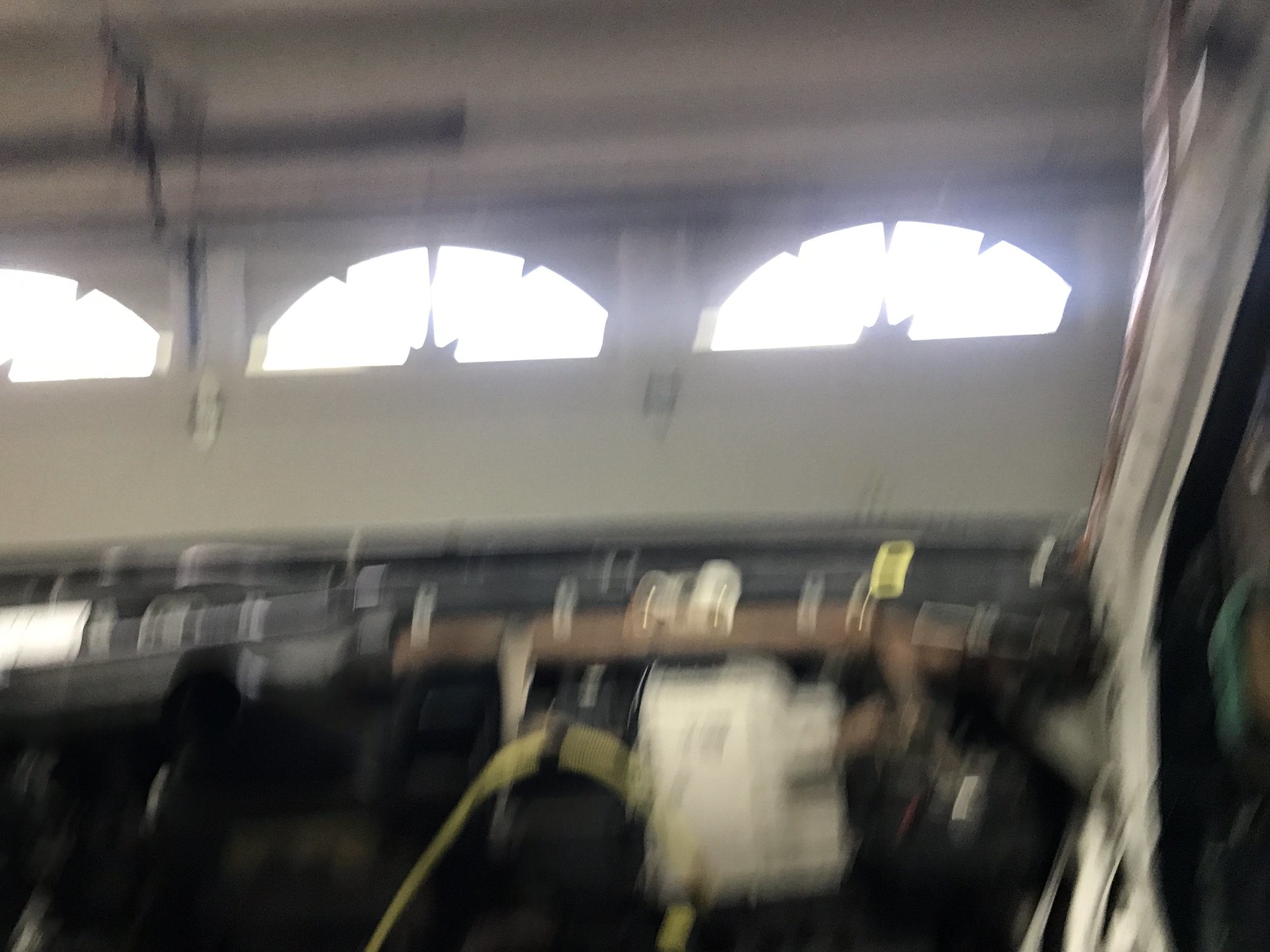This image appears to be taken inside a garage, focused on an inner garage door identifiable by its distinct arch-shaped windows. There are two and a half windows visible in the frame, with the far left one partially cut off. The door itself is painted white. Above it, some pieces of equipment are visible, suspended or mounted. The foreground is dominated by what seems to be the underside of a vehicle, though the blurriness of the image makes it difficult to determine specific details. A white item with a yellow cable, which could be either connected to it or positioned in front of it, adds to the scene's complexity. Additionally, there is a rust-colored pipe, possibly part of a muffler, situated just above this item. The overall image is somewhat unclear, adding a mysterious and cluttered vibe to the scene.